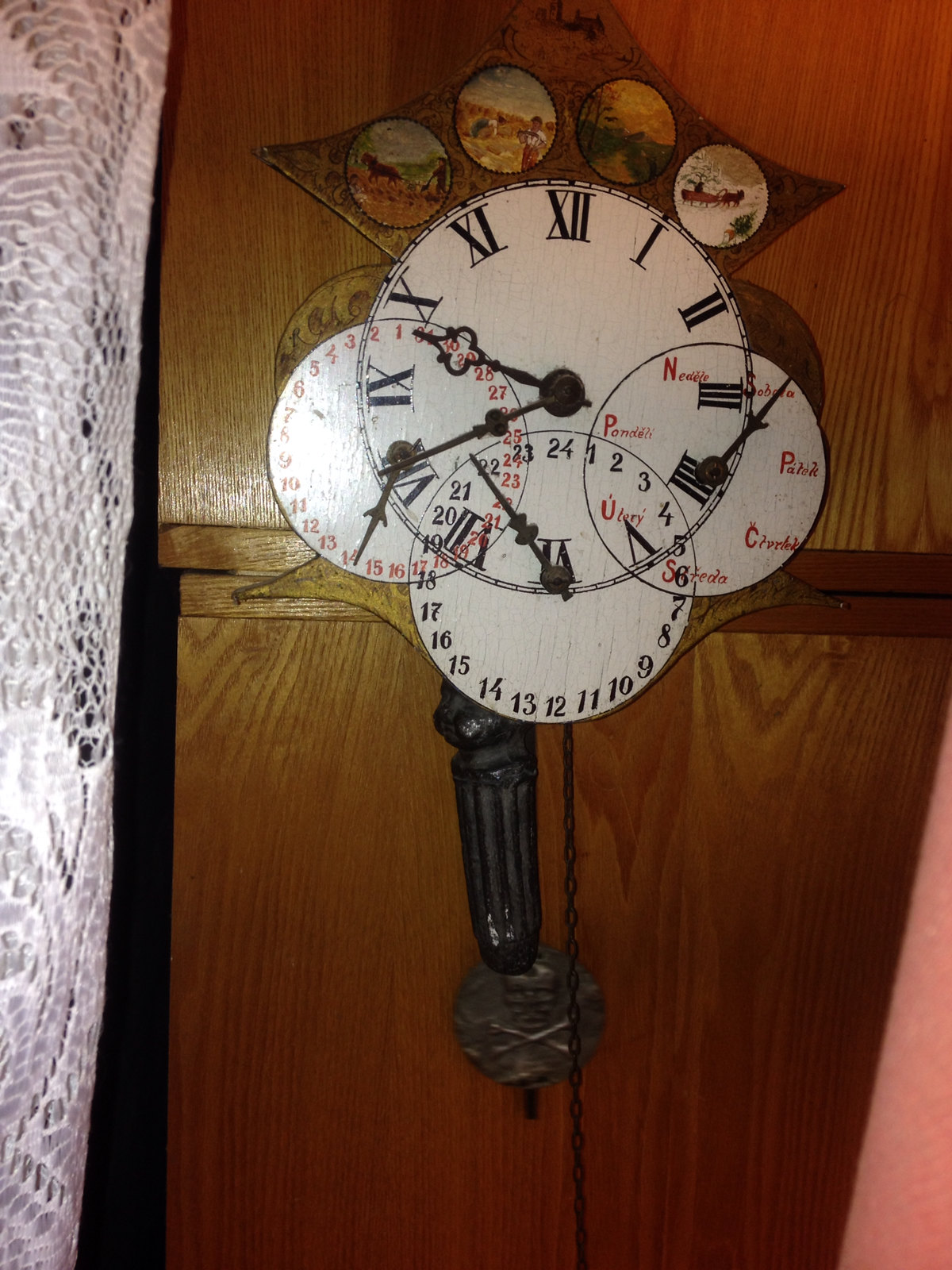A richly detailed and nostalgic image depicts an antique clock mounted on a paneled wall. To the right, a delicate white lace curtain encroaches about an eighth of the way into the picture, adding a touch of elegance. The top of the clock features a star-shaped embellishment adorned with four distinct illustrations representing the changing seasons. Spring showcases a farmer diligently plowing a field, followed by a summer scene of two individuals working together in the field. Autumn is subtly depicted with fall leaves adorning a tree, while winter portrays a horse-drawn sleigh gliding through the snow.

The clock itself is a masterpiece of design, comprising four concentric circles. The primary clock face is distinguished by traditional key-shaped hands and Roman numerals, indicating the time as 8:35. Adjacent, the first inner circle on the left displays text in red, written in an undetermined language. 

The second circle, located at the bottom of the clock, functions as a 24-hour clock, currently pointing to the 22nd hour, corresponding with 10:35 PM. The third inner circle presents a unique 30-minute timer that appears to operate counterclockwise, with its hand resting on the 14th minute mark. 

Completing this intricate composition is a piece of dangling metal, likely a chime, adding to the clock's vintage charm and hinting at its potential for melodic sound.